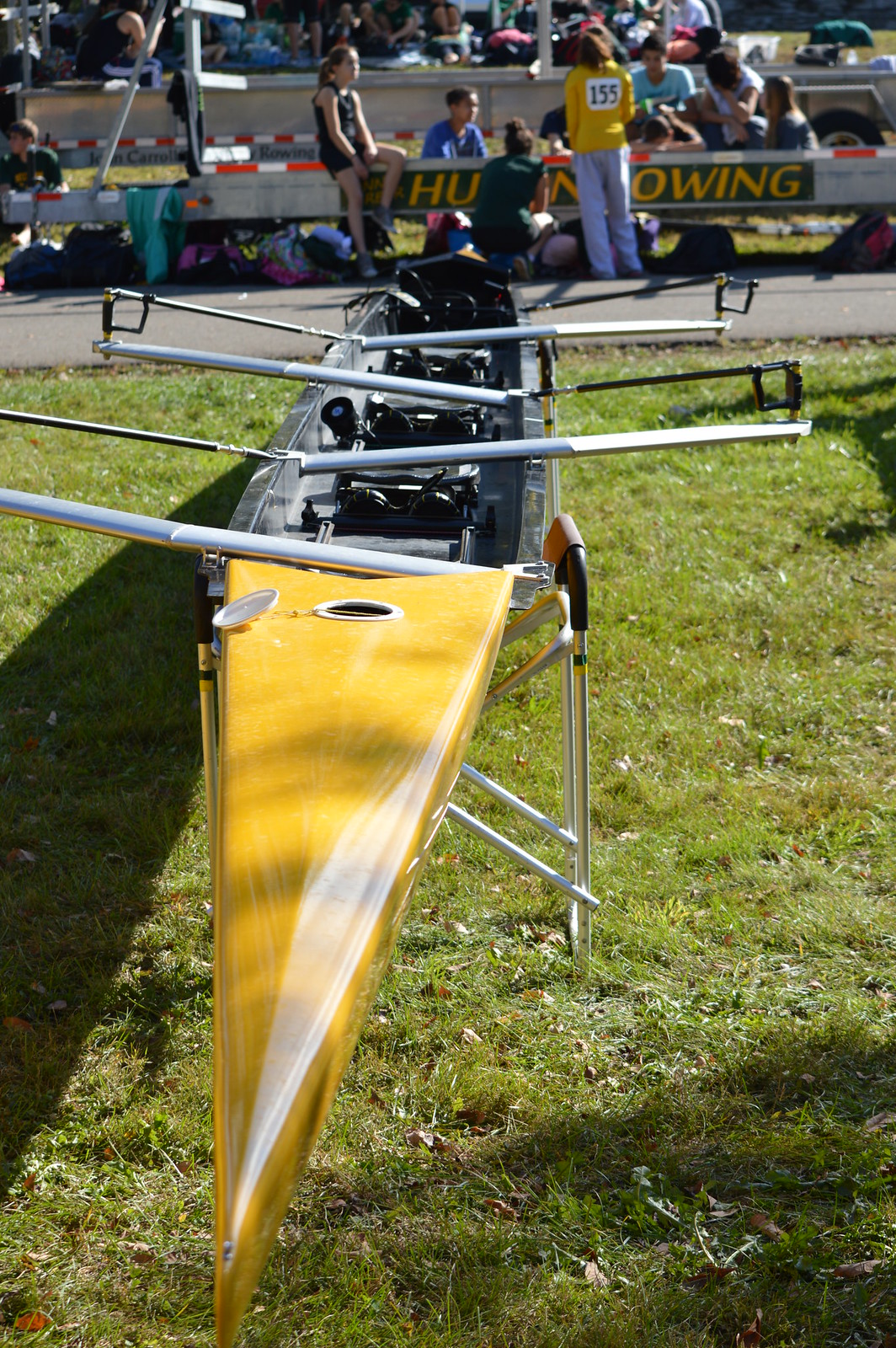The image captures a vivid scene at a rowing competition on a clear, sunny day. Dominating the foreground is a long, pointy yellow kayak, resting on a stand positioned on a grassy area. The kayak is designed for three individuals, with metal oars attached along its sides for each rower. In the middle ground, a young girl with red hair, dressed in black shorts and a black tank top, sits atop a trailer. Nearby, another person with long red hair and a yellow long-sleeve shirt, bearing the number 155 on their back, stands facing away from the camera. The background reveals a bustling atmosphere with numerous participants and spectators. Several individuals, identifiable by the numbers on their backs, are situated near a concrete area next to a trailer, indicating their involvement in the competition. A variety of people can be seen sitting or standing by a barrier that runs along the grass, extending towards a waterway visible in the distance. The crowd includes what appears to be parents and audience members, suggesting a lively and well-attended event.